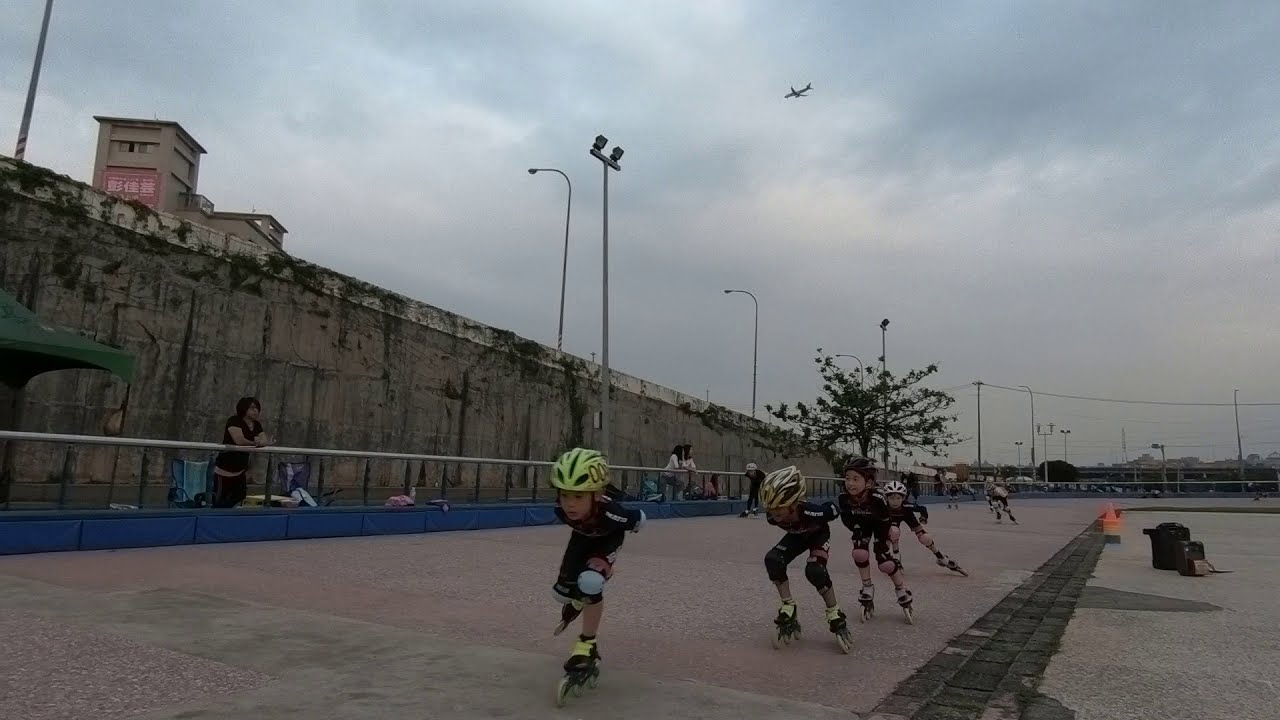In this detailed image, six young rollerbladers are gliding in a line on a concrete oval track, navigating its intricate details with precision. The front skater is distinguishable by a light green helmet, a black suit, and light yellow accents on their skates. Following closely behind is a skater adorned with a mostly black helmet streaked with hints of yellow, and another skater clad in a black suit and black helmet. Further along the line, one skater sports a white helmet, and the other two skaters, though visible, are too distant to discern clearly. 

The track itself comprises a primary gray concrete surface interspersed with amber sections, hinting at wear or design variations. Flanking the left side is a barrier where onlookers are leaning, marked by a white pole atop a chain-link fence lined with a blue tarp at the bottom. Beyond this fence, a verdant wall, cloaked in moss and brownish streaks, stretches out, contributing to the natural enclosure of the area. A substantial, multi-story brown building towers in the distant left background, casting a shadow over the track.

Illuminating the scene, lights are strategically placed above the rollerbladers and at the back right-center, casting a spotlight on their path. Overhead, power lines drape across the cloudy, grey sky, accentuating the overcast ambiance. An airplane is visible in the sky, flying towards the left, adding dynamism to the static elements below. This photograph captures a vivid and bustling scene of young athletes fervently engaged in their sport with spectators closely watching their every move.